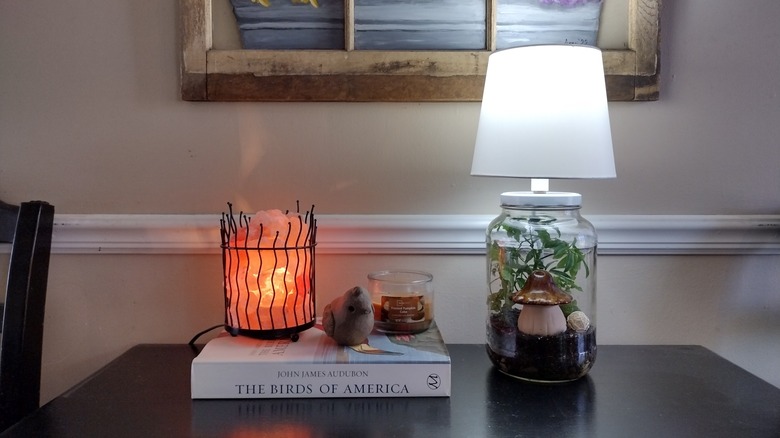The photograph captures a cozy, eclectic interior setting featuring a dark espresso-colored table adorned with several interesting objects. Central to the tableau is a prominent book titled "The Birds of America" by John James Audubon, its large white spine clearly visible. Atop this book rests a unique mood-enhancing salt lamp, glowing with a warm pink to orange hue, surrounded by black, wavy, cage-like lines. Beside it, there's an unlit candle and a small bird decoration, possibly a statue or a stuffed toy.

Further to the right, a fascinating lamp with a jar as its base catches the eye. The transparent jar contains an arrangement of shells, leaves, plants, and a ceramic mushroom, all crowned by a white lampshade. This lamp adds an earthy, whimsical touch to the warm and inviting setting.

In the background, a piece of artwork depicting a serene beach scene adds depth and charm to the space, while the bottom of a window with a worn wood frame is partially visible, contributing to the homey, tranquil atmosphere. The table surface is cluttered in an artful way, each item contributing to a sense of intrigue and comfort in this personalized home interior.